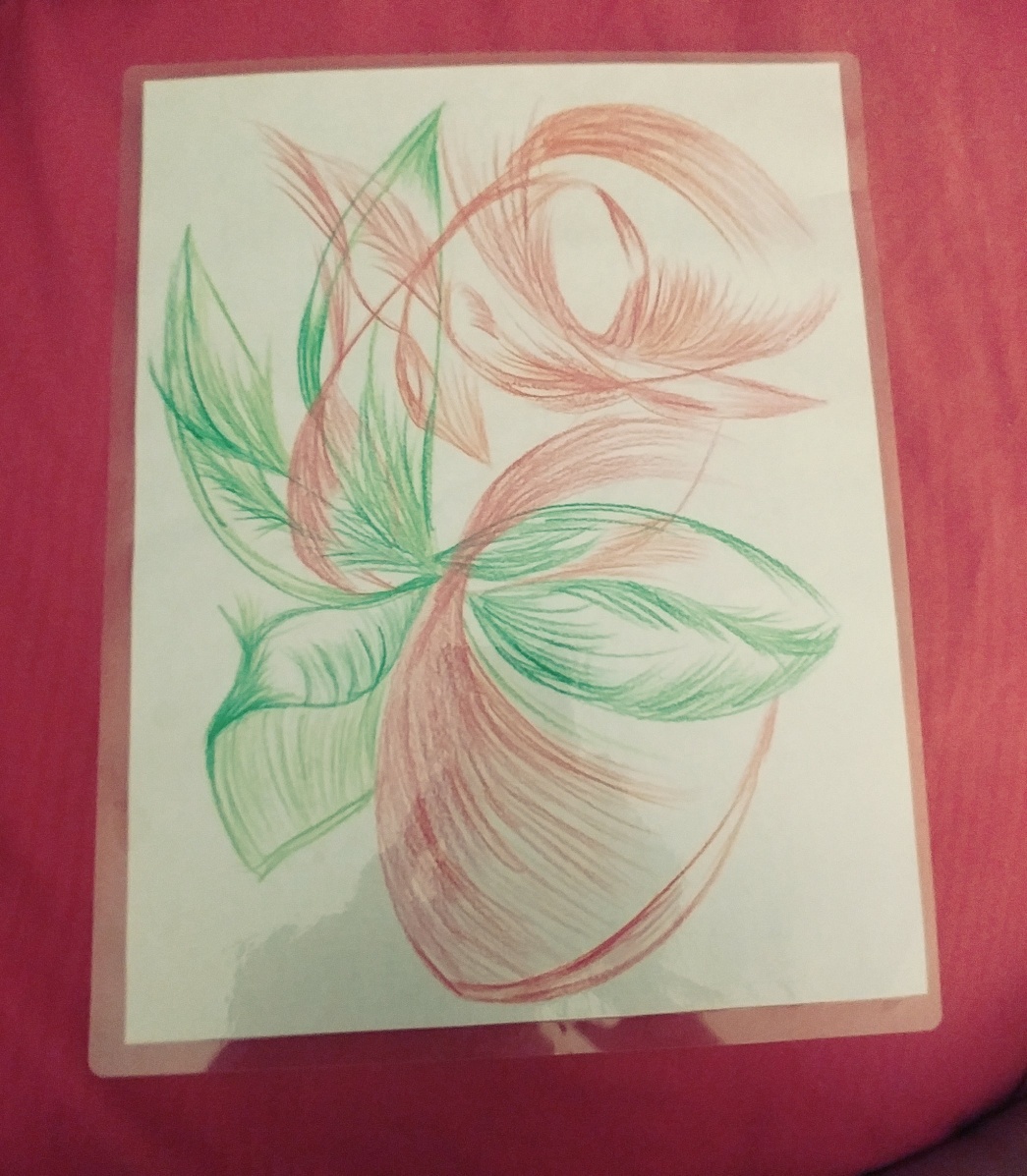A striking image features a background of vibrant red fabric, creating a rich, luxurious backdrop. In the foreground, a laminated or plastic sheet showcases an intricate drawing rendered in colored pencils. The artwork primarily depicts a plant with dynamic, swirling structures. Reddish-brown leaves emerge from the bottom right, spiraling upwards and to the left before coiling back towards the middle and extending up to the right. Alongside them, verdant green leaves weave intricate, vein-like patterns, branching out in a natural yet stylized manner. The leaves on the left side of the drawing curl upwards gracefully. The entire scene is characterized by multi-layered, sketch-like swipes that add depth and motion to the botanical illustration.